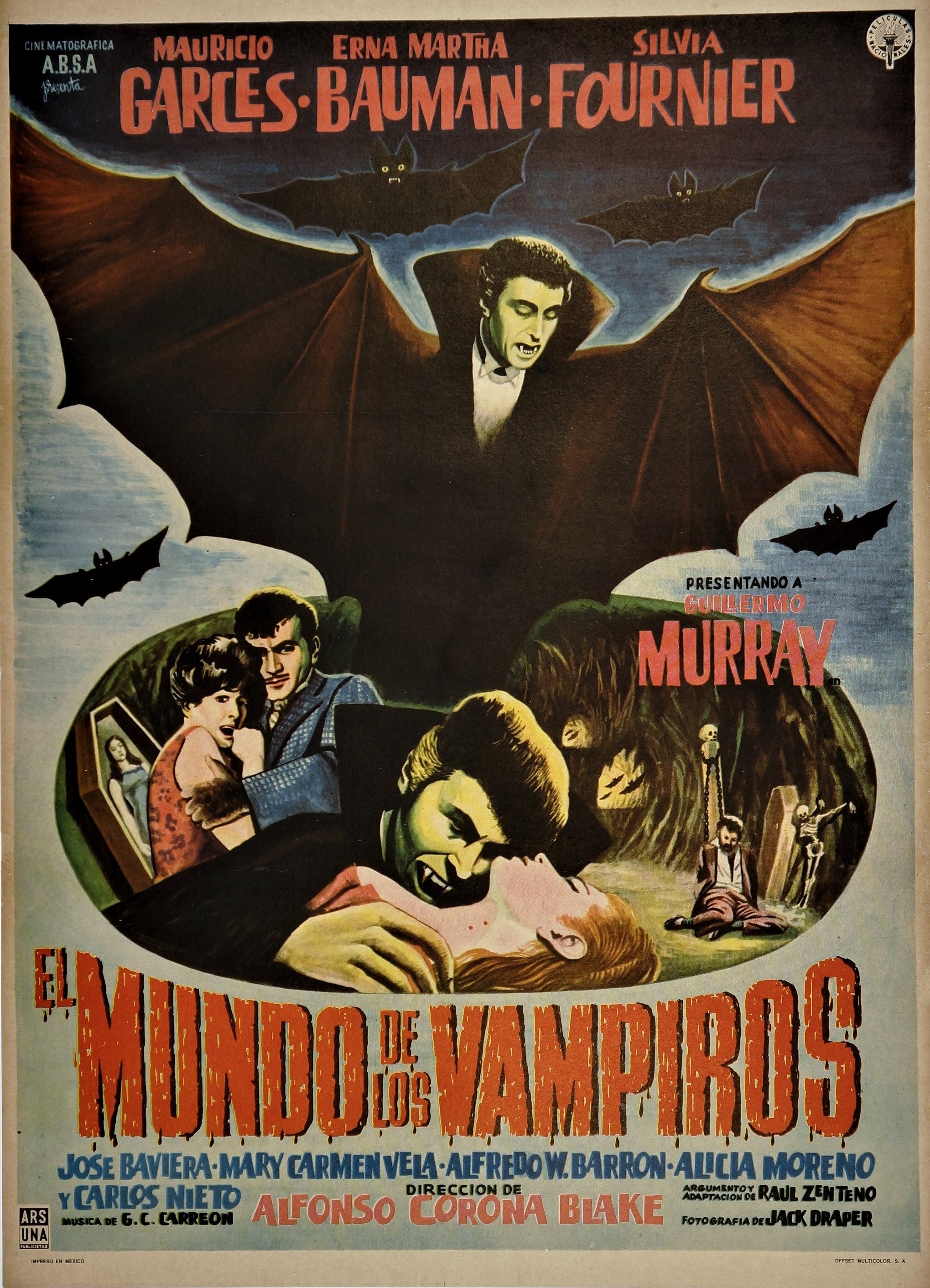This is a vintage movie poster for "El Mundo de los Vampiros" (The World of the Vampires), a Spanish film. Dominating the poster is an artwork of Dracula, portrayed with bat wings, green skin, tall black hair, and fangs prominently displayed. He is dressed in a black ensemble with a white shirt, and he's gazing menacingly downwards. Surrounding him are eerie black bats with bright yellow eyes. Below, in a circular inset, Dracula is depicted with his fangs poised to bite a blonde woman with pale skin, who appears unconscious. Around them, onlookers are shrieking in horror; one, resembling a wolfman with shaggy hair and hairy hands, dons a blue suit. Nearby, a brown coffin lies open with a woman inside. The poster also includes three different scenes within an oval space: a woman in a coffin, a frightened couple embracing, and a man held captive in a cave with skeletons. The movie title, "El Mundo de los Vampiros," is inscribed in red, dripping text, adding to the gothic and terrifying aesthetic. The poster also lists the names of the cast: Mauricio Garcias, Erna Martha Baumann, Sylvia Forner, Guillermo Murray, Jose Baviera, Mary Carmen Vela, Alfredo W. Barron, Alicia Morenzo, Carlos Nieto, with direction by Alfonso Corona Blake, Raul Zenento, and Jack Draper.